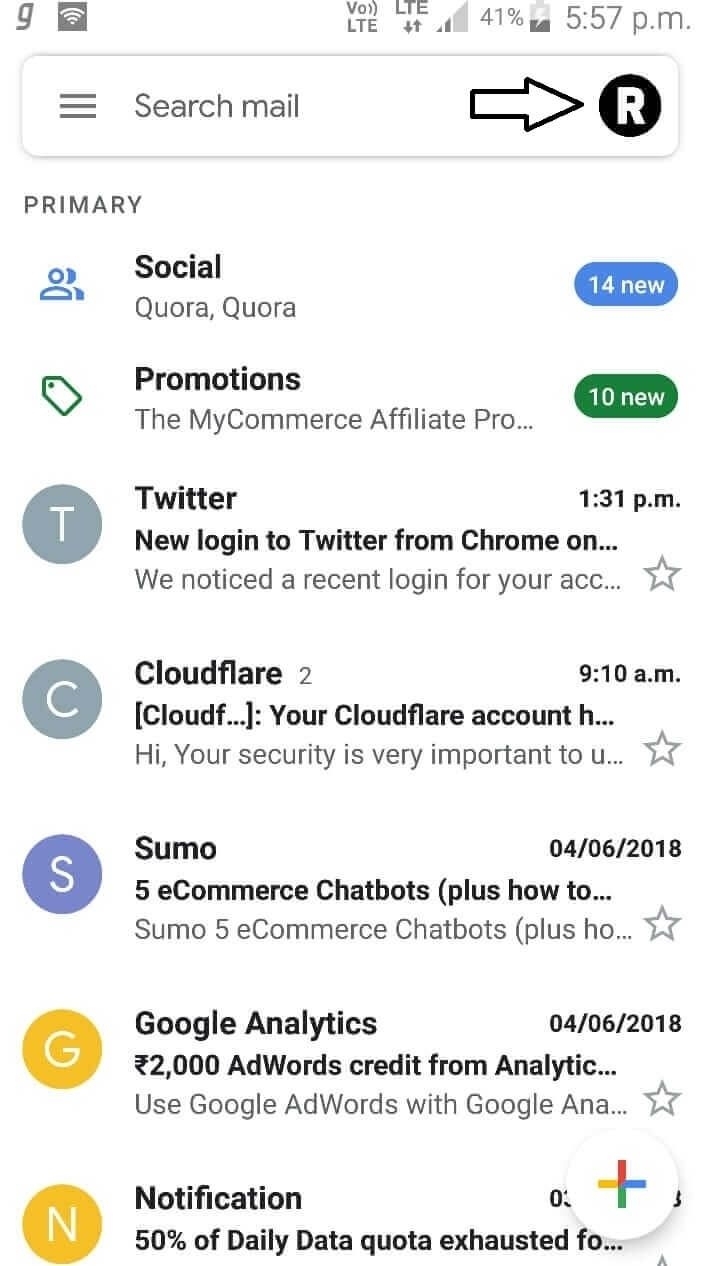This image is a screenshot of an email interface on a cell phone. At the top of the screen, visible symbols and indicators are present on the upper right and upper left, denoting signal strength, battery status, and other notifications. Directly below these symbols is a search bar with the placeholder text "Search mail." Inside this search bar, on the far right, is a black circle containing a white capital "R." Also located in the search bar is a black outlined arrow with a white center.

Below the search bar, the screen displays the word "Primary," indicating the selected email tab. The "Primary" tab lists seven items, arranged one beneath the other. Here is a detailed breakdown of each item:

1. The first item is categorized under "Social," showing two entries labeled "QUORA, QUORA". To the right, it indicates "14 new" messages.
2. The second item is under "Promotions," specifically noting the "MyCommerce Affiliate Program," with "10 new" messages.
3. The third item highlights notifications from "Twitter," specifying a "New login to Twitter from Chrome," with a timestamp of 1:31 PM.
4. The fourth item is a notification from "Cloudflare," marked with a timestamp of 9:10 AM.

This detailed description captures all visible elements and provides context for each item in the email interface.